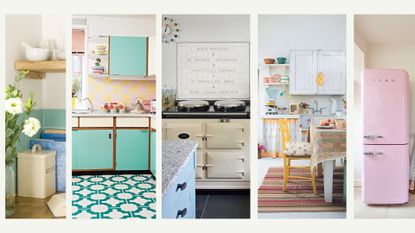The image is a composite of five distinct rectangles, each depicting different segments of a home. Starting from the left, the first rectangle shows what appears to be a small laundry area with a beige rectangular container, a potted plant with large white flowers, a taller blue object possibly a basket, and a shelf bearing what looks like a mortar and pestle. The second rectangle features a kitchen with blue and white circular-patterned floor tiles, blue cabinets topped by white drawers with wooden trims, a white kettle on the counter, and a white and yellow wallpaper background. There is also a glimpse of a window.

The third rectangle seems to be a multifunctional room, possibly part of the kitchen or a nearby area. It has blue drawers in the foreground, a white cabinet with what might be a stove, and a colorful clock in the top left corner. Scattered on a benchtop are some black shapes and a white board with illegible writing.

The fourth rectangle is likely a dining or playroom area, characterized by a multicolored mat on the floor with a yellow chair, a white table draped with a colorful tablecloth, and a variety of cabinets with some open, displaying assorted items including red and blue crockery. Yellow-handled cabinets are also visible, contrasting the white walls and floor.

The final rectangle is the simplest, showcasing a retro-style pink refrigerator with chrome handles, situated in a beige room. This composite image effectively captures various domestic spaces, each room providing a snapshot into the home's diverse and colorful décor.